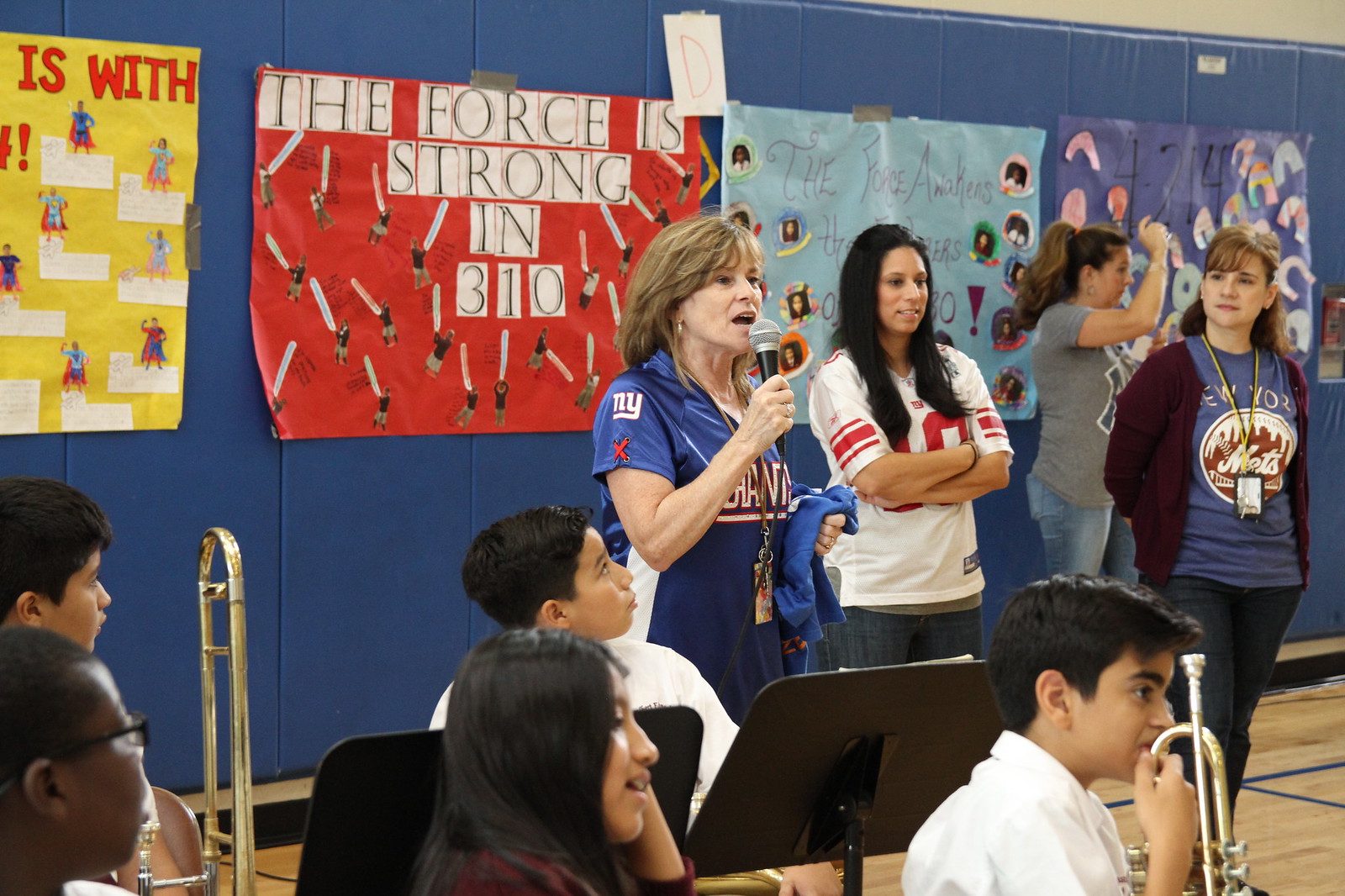The photograph captures an indoor middle school music event, held in the gymnasium, as evident from the wooden floor with blue basketball markings visible in the lower right corner. The backdrop consists of a plain black wall adorned with student-made construction paper signs, one prominently reading, "The Force is Strong in 310."

Three adult women stand near the center right of the image, each sporting sports jerseys: the central woman, possibly a teacher or coach, is addressing the audience with a microphone and is wearing a New York Giants jersey. To her right is a young woman with black hair wearing a white and red NY jersey, and further to the right stands another young woman with light brunette hair in a burgundy cardigan and a New York Mets shirt.

Situated in the bottom section of the image are several young students, seated with music stands in front of them. Some hold brass instruments, such as a trombone and a trumpet, though the instruments of others aren't visible. The overall image is vibrant with colors including blue, red, white, brown, black, gray, pink, yellow, gold, tan, and orange, encapsulating the lively atmosphere of this school event.